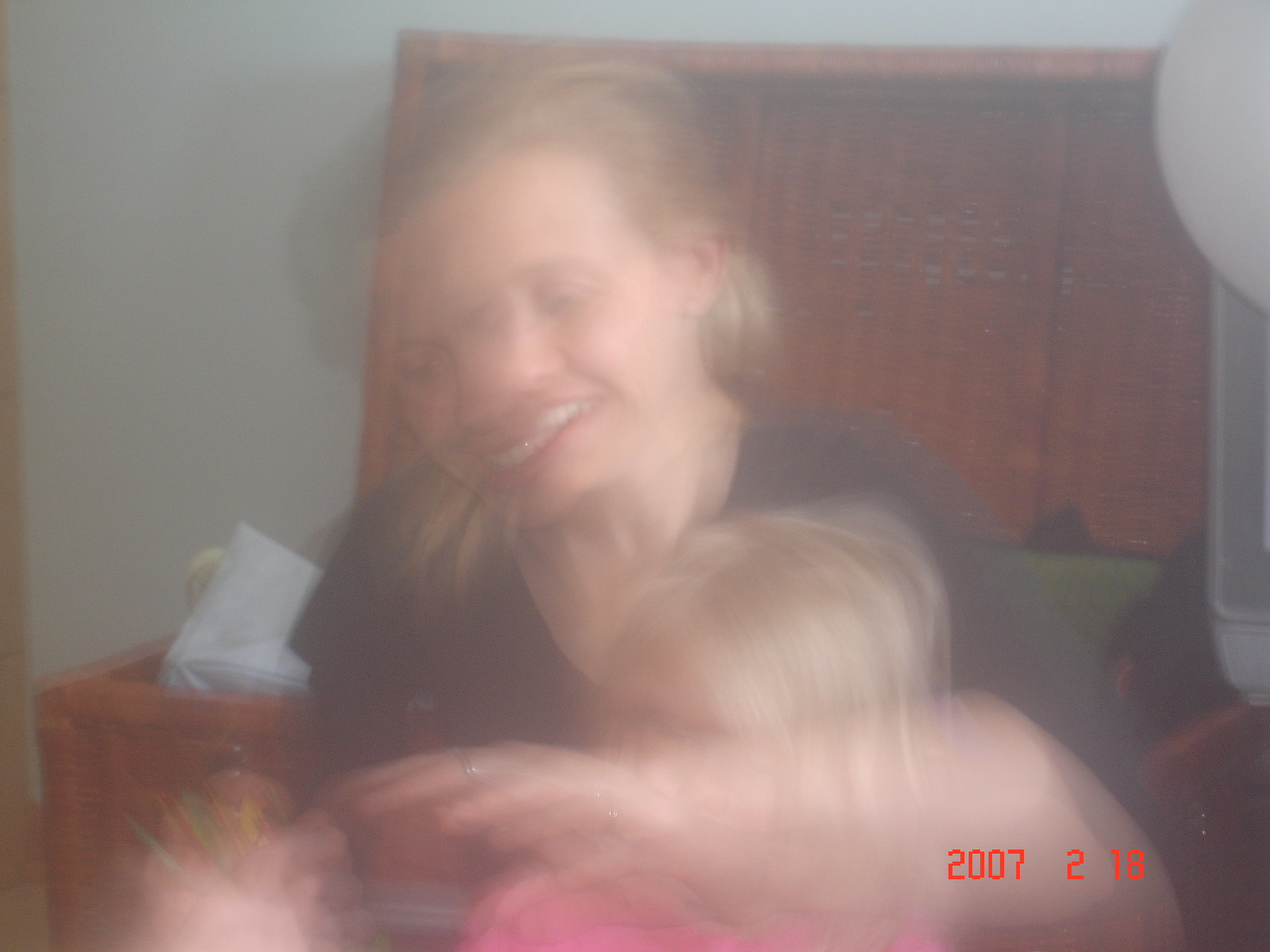In this blurry photograph, a woman with shoulder-length blonde hair, dressed in a dark blue short-sleeved shirt, is captured smiling and looking down affectionately at two small children. The image appears to be taken in multiple frames, giving the woman an ethereal appearance with three faces at different angles. 

On her left side, there's a barely distinguishable child with dark brown hair, represented by a head-shaped blur. On her right, the more defined child, with medium-length blonde hair, wears a bright pink or neon sweatshirt. The woman has her arm protectively over this child.

The setting seems to be a cozy indoor environment, possibly a restaurant or living room. Behind her, there is a wood panel and what appears to be the back of a green couch. On her left, a wooden box is visible, with a couple of tissues peeking out, adding to the homey atmosphere of the scene.